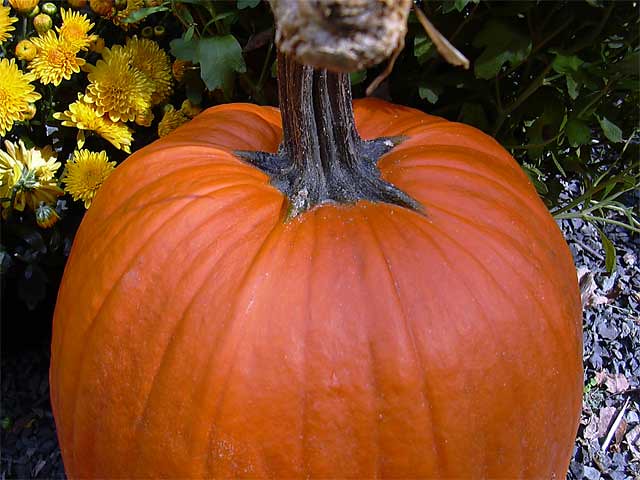In this square image, a prominently round and symmetrical orange pumpkin takes center stage, filling up nearly the entire frame. The pumpkin features characteristic vertical lines and ridges, and is topped by a short, dark brown-gray stem. Surrounding the pumpkin, the scene is adorned with various plants and flowers. To the left of the pumpkin, there are several vibrant yellow mum flowers, providing a burst of color. Above these flowers and extending toward the center, green leaves contribute to the lushness of the setting. On the right side of the pumpkin, light purple flowers or plants add an additional layer of visual interest. The lower part of the image, particularly towards the bottom left corner, is darker, with only a few leaves discernible in the shadowy area. The background towards the right also darkens, but green leaves and stalks are still visible, protruding into the scene. Overall, the image captures a harmonious autumn tableau with the pumpkin as the focal point, framed by a rich variety of foliage and flowers.